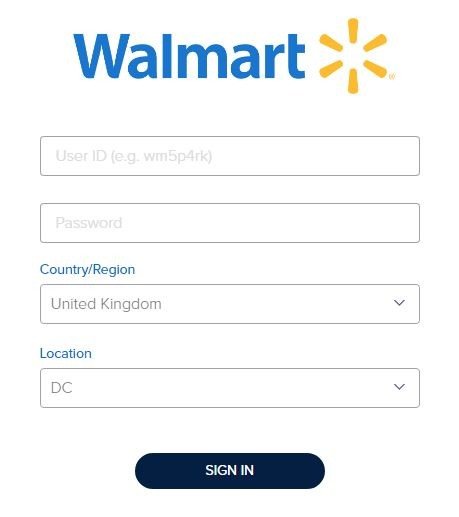This image captures a login page for Walmart, set against a clean white background with minimal text and imagery. Dominating the top-middle section of the page is the word "Walmart" in a distinctive blue font, juxtaposed with the iconic yellow Walmart logo to its right. Directly below this, a rectangular text box bordered in black contains lighter, less legible gray font, displaying "User ID (EGWM5 P4RKN)". 

Underneath the user ID input field, another rectangular text box with a gray border awaits the user's password, indicated simply by the word "Password". 

Further down, in blue text, the labels "Country/Region" and "Location" are presented against the white background. The "Country/Region" label is followed by a text box that reads "United Kingdom," while the "Location" label is succeeded by a text box containing the capitalized letters "ABC."

At the very bottom center of the page, a dark blue rectangular button prominently displays the phrase "SIGN IN" in bold white capital letters, inviting users to proceed with their login credentials.